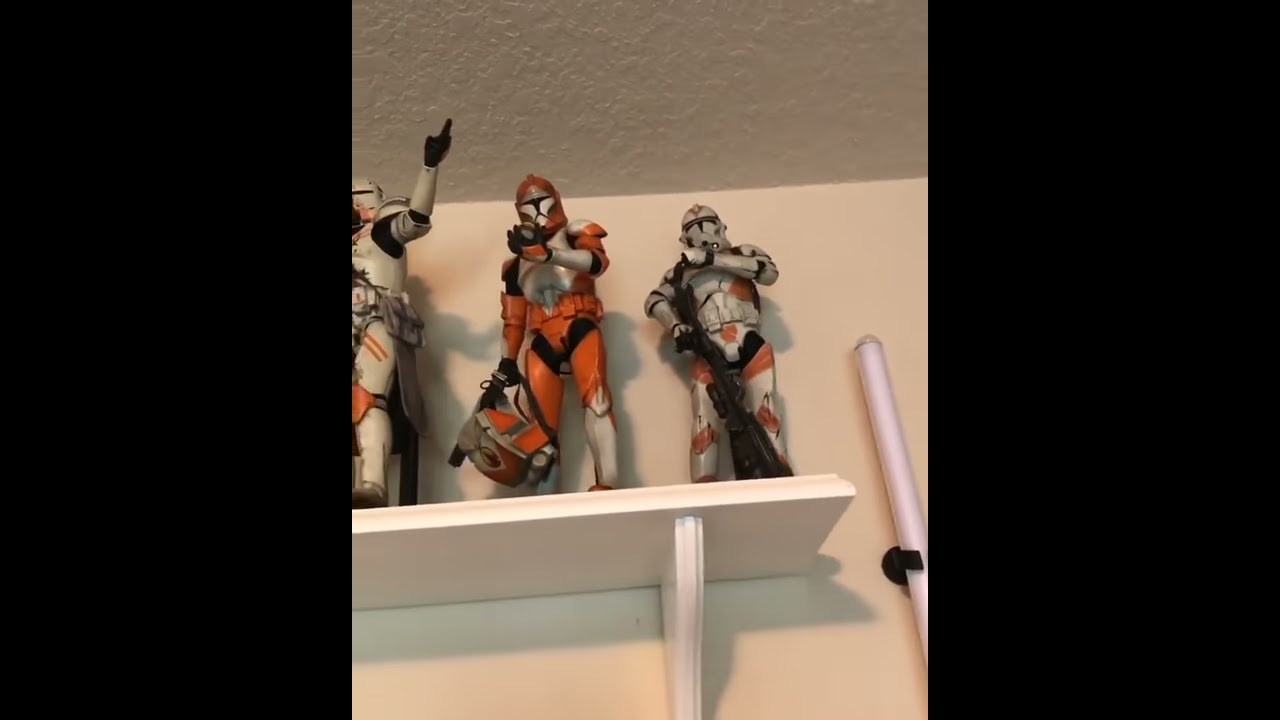The image captures a screen grab from a social media video, showcasing a high-floating shelf near the ceiling of a room. The shelf prominently displays three Star Wars collectibles, specifically Stormtrooper figurines wearing armor from the recent films. The figurines are arrayed as follows: the left one is white with orange accents, and has its arm raised with a black glove, pointing upwards. The middle figurine is primarily orange with white highlights. The right figure is similar to the first but inversely colored, being mostly orange with white accents, and appears to be holding a weapon. Mounted on the wall to the right of the shelf is a model lightsaber. The scene also features a white ceiling with a distinct texture pattern and a glimpse of the whitish textured wall below it. Two black rectangular shapes flank the higher part of the frame.